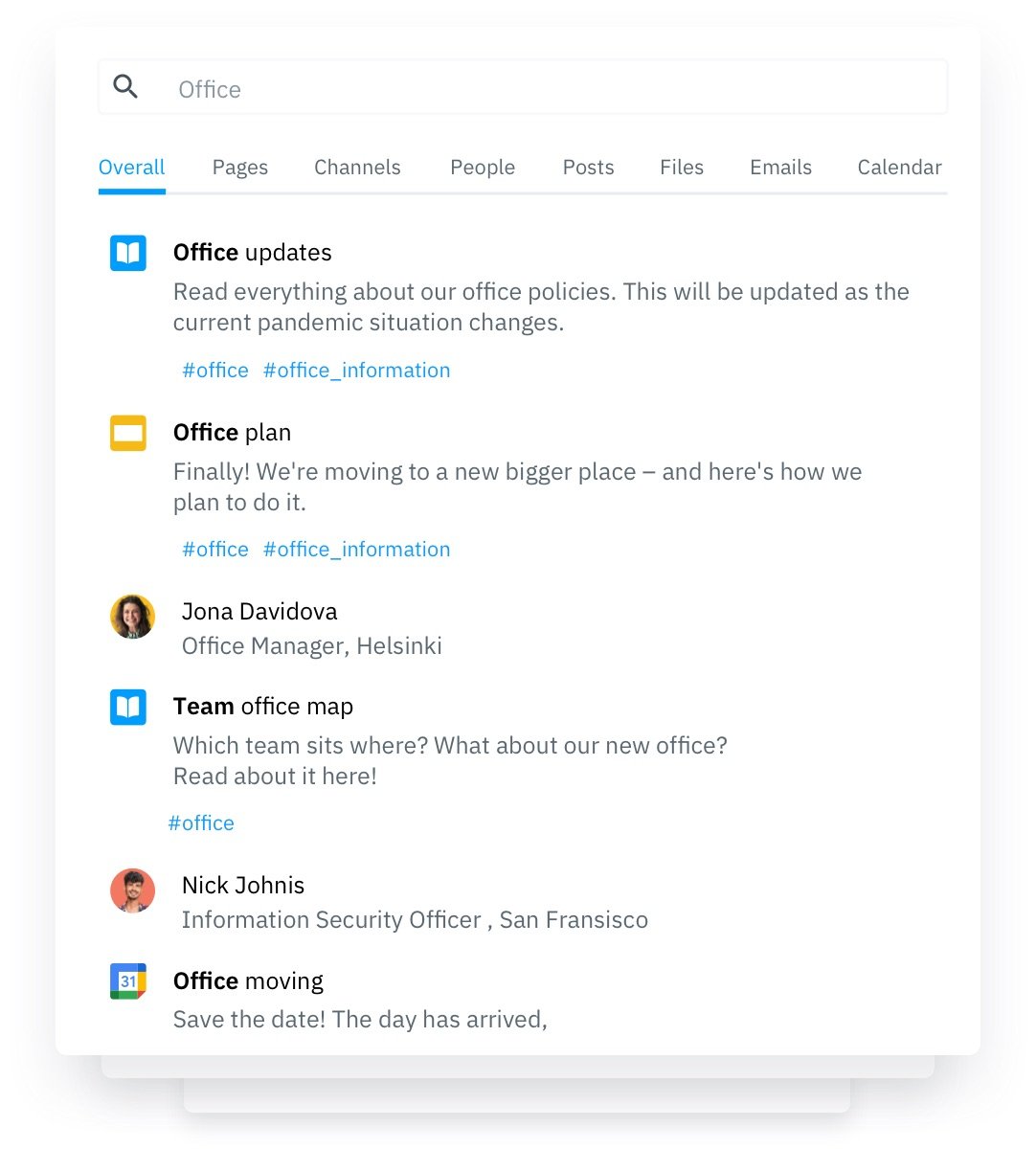In the image, we have a screenshot set against a solid white background. In the upper left corner, there is a gray magnifying glass icon next to the word "Office." Below this, a row of tabs is displayed, from left to right: "Overall," "Pages," "Channels," "People," "Posts," "Files," "Emails," and "Calendar."

Underneath these tabs, there is an icon of a book with the label "Office Updates," accompanied by the text: "Read everything about our office policies. This will be updated as the current pandemic situation changes." This section includes the hashtags #office and #office_information.

Further down, there is another section titled "Office Plan," with the text: "Finally, we're moving to a new, bigger place, and here's how we plan to do it." This section also includes the hashtags #office and #office_information.

At the bottom of the image, there is a photograph of a woman named Jonah Davidova, identified as the Office Manager in Helsinki.